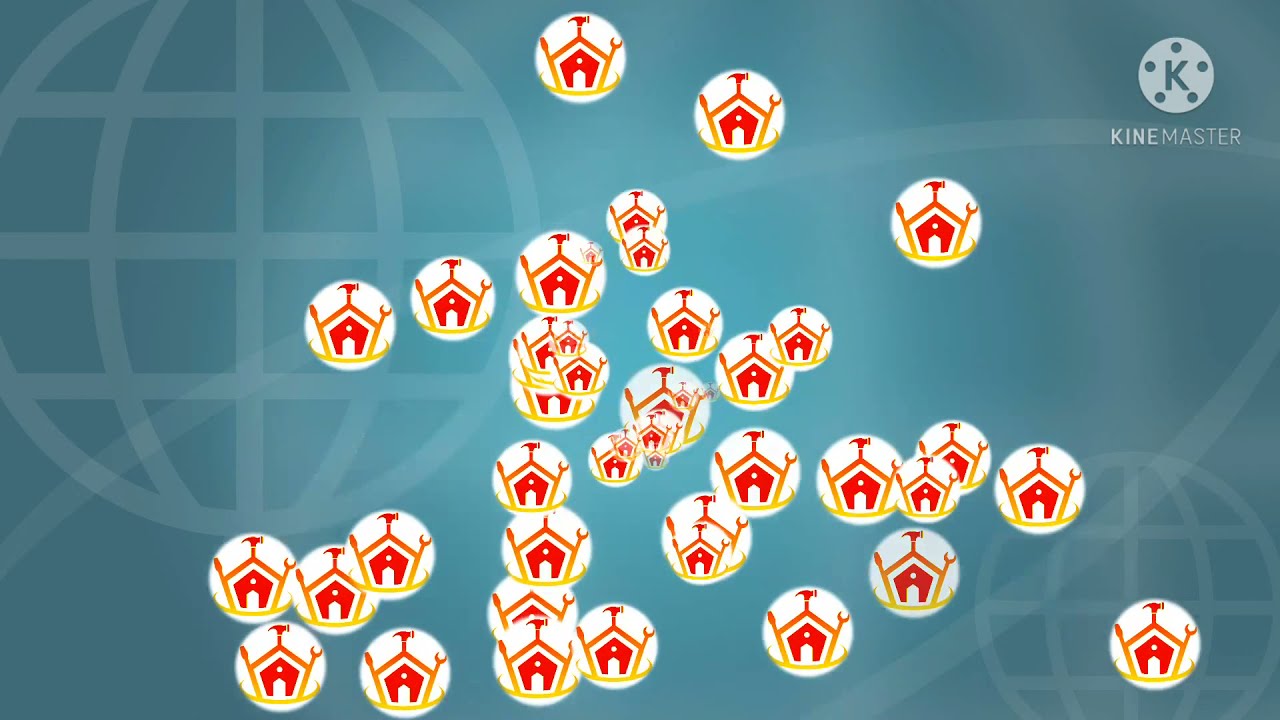This web graphic for KineMaster features a detailed and vibrant illustration against a gradient aqua blue background. Prominently, the KineMaster logo with a white encircled 'K' bordered by blue dots is displayed in the upper right corner, with the brand name "KINEMASTER" written underneath. The background also includes globe-like graphics showing meridians and latitudinal lines, positioned in the upper left and bottom right corners.

The central and lower portions of the image are scattered with about 30 smaller white circles. Each circle contains a red, geometric house icon. The house features a simplistic design with white roof extensions at three corners: a hammer at the central peak, a crescent moon-like shape on the right, and another tool on the left. There is also a golden swirl at the bottom of the house icon.

Overall, the image blends elements of technical illustration with vibrant, clean design elements, enhanced by likely Photoshop filters and effects to create a cohesive and dynamic visual representation of the KineMaster brand.